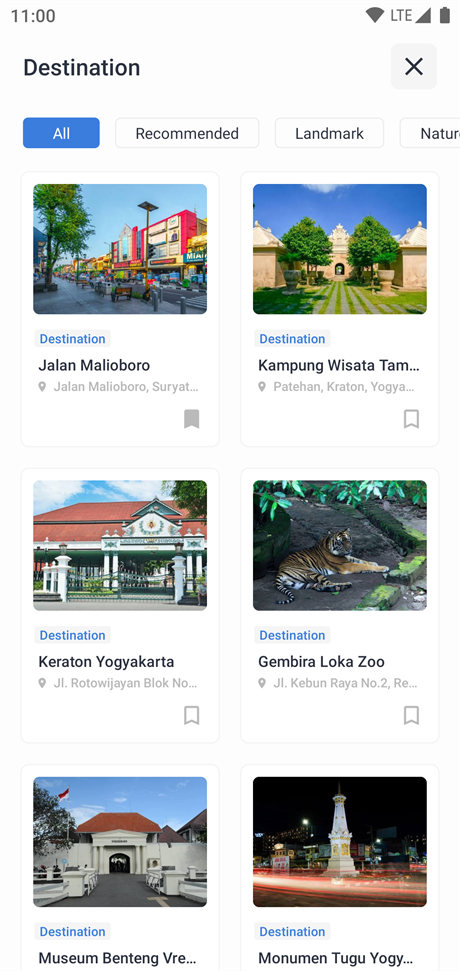The screenshot showcases a mobile app interface. At the top right corner of the screen, the time is displayed as 11:00. Next to the time, there are icons indicating full-strength Wi-Fi, LTE with 5 bars, and a fully charged battery. 

The main content of the app page starts with a top-left section where the word "Destination" is written in a sans-serif font and capitalized, followed by an 'X' icon on the left for closing. Below this title, there are four horizontally aligned navigation links. The links are labeled "All," "Recommended," "Landmark," and the last one is partially truncated but appears to start with "Nature."

Beneath these navigation links, the app displays six high-resolution thumbnail images of various destinations. Each thumbnail includes a locator icon and a brief description:
1. Destination with a grey marker flag.
2. Kampong Wisata Tam... located at Patihan, Traton, Yogyakarta.
3. Keraton Yogyakarta.
4. Destin Kin, J.I. Rotojohn Block No...
5. Jimbira Lake, Lokazu located at Jail Keburn, Raya No. 2 RE...
6. Museum Bentang Berry...
7. Monument Tugu Yogi...

These images feature single places of interest or specific buildings, and the background of the app page is white.